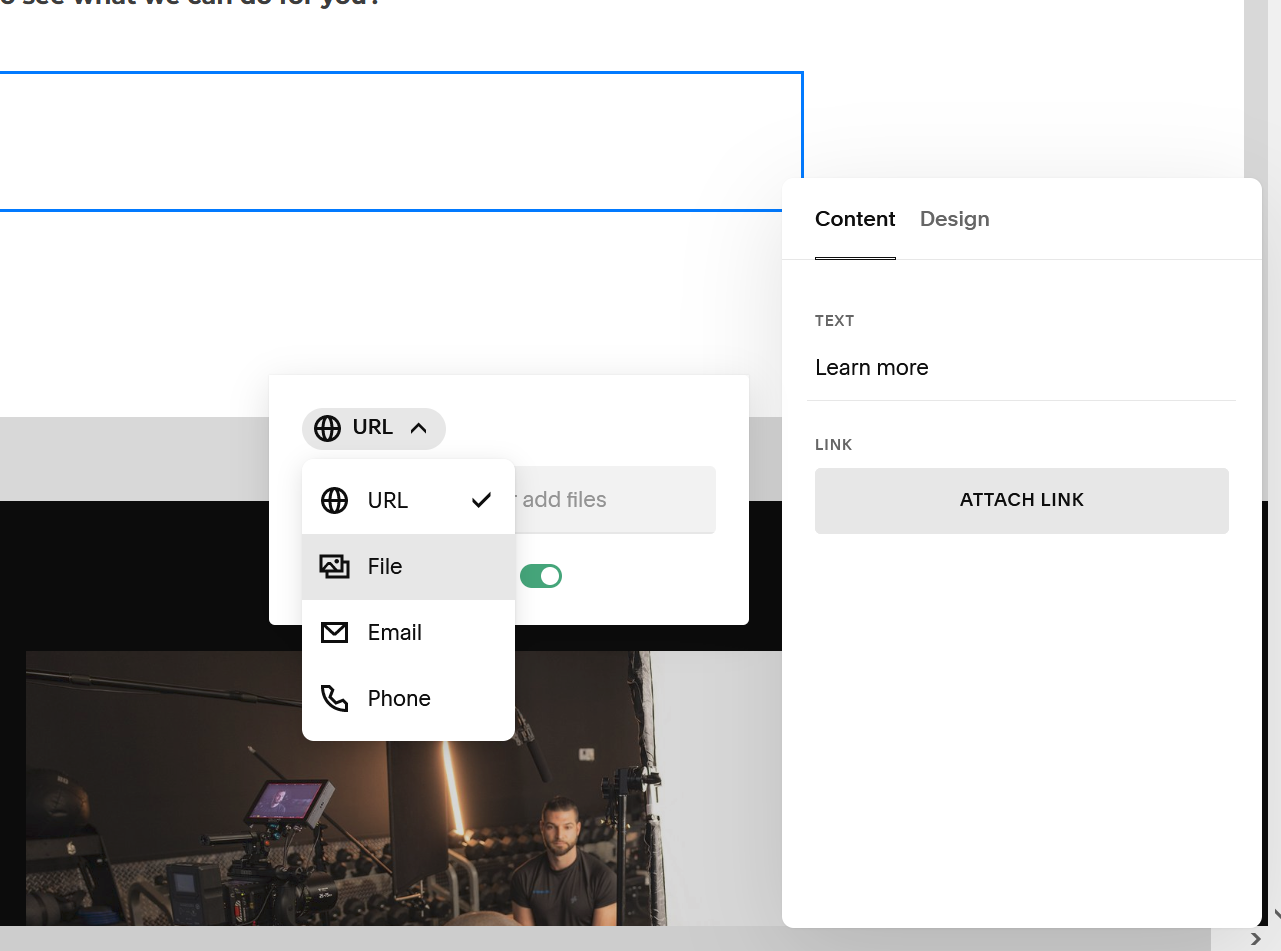This image is a portrait-oriented screenshot of a web design interface, possibly part of a content management system where editing is taking place. Although slightly cut off, several elements are discernible. 

The background is predominantly white. At the very top, there is partially visible text, with the last word ending in "you!" before being cut off. Below this, there is a significant amount of white space followed by a blue rectangular box extending horizontally across the screen, also exhibiting white space within it.

On the right side of the screen, there is a vertical white pop-up box rooted at the bottom and featuring two selectable options: "Content" and "Design." The "Content" option is highlighted in bold and underlined, emphasizing its selection. Further down, a borderline is noted underneath which displays options including "Text," "Learn More," "Link," and "Attach Link."

Adjacent and below this is another pop-up box, providing additional selection options which include an entry labeled "URL" accompanied by an icon and a checkmark, along with other choices like "File," "Email," and "Phone."

At the bottom of the interface is a photo depicting a man seated in what appears to be a gym. In the photo, an exercise bike screen and some weights are visible in the background, providing context for the setting.